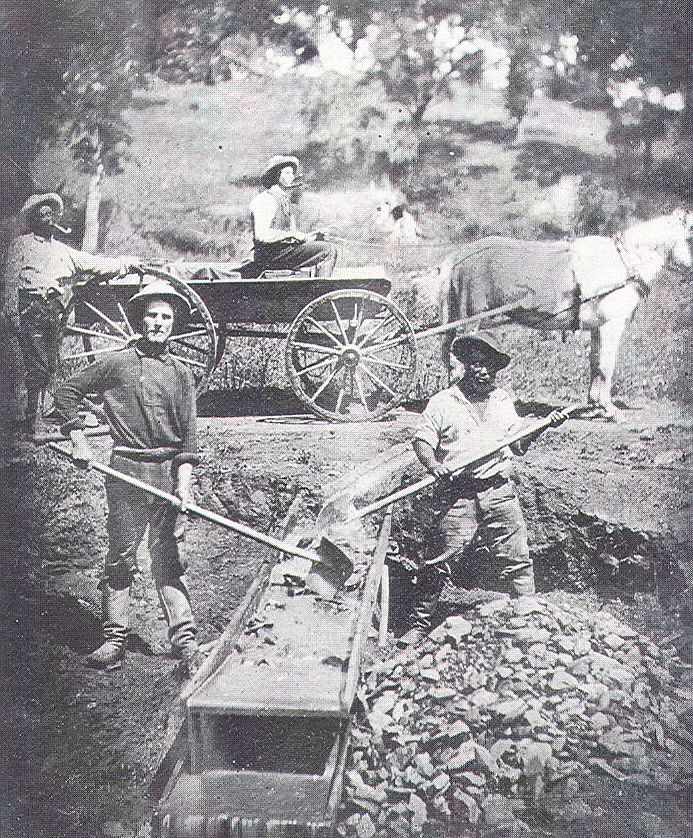This vertical, rectangular, black-and-white photograph appears to be from the early 20th century, possibly the 1920s to 40s. It depicts a group of people engaged in either construction or mining work. In the foreground, two men, each holding a shovel, stand on either side of a prominent black woodblock structure situated on dirt ground. The man on the left, dressed in jeans, a white shirt, and a hat, stands near a pile of rocks, while the man on the right, in darker clothing, also wears a hat. Behind them is a horse-drawn wagon with two large wheels, containing a woman in a hat, possibly holding a corncob pipe. A white horse is harnessed to the wagon, facing right. Another man, in a white shirt and dark pants, stands at the back of the wagon with his hand on one of the wheels. The background is somewhat grayed out, evoking an old-time feel, with faintly visible trees lining the top of the image, enhancing its vintage atmosphere.